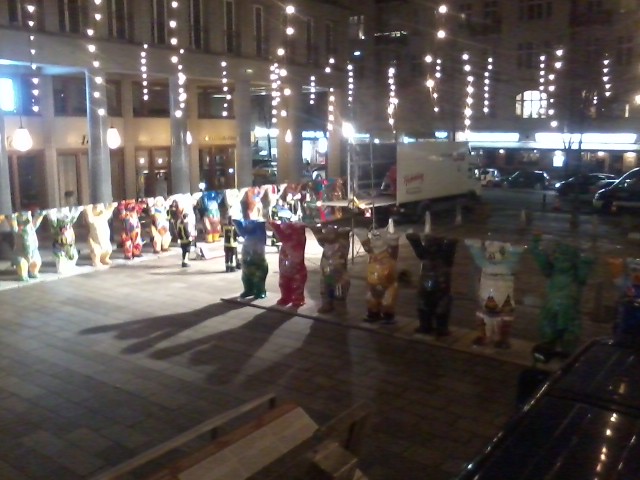This nighttime cityscape photograph captures a vibrant courtyard installation nestled beside a hotel-like building adorned with white piers. The main attraction is a series of multicolored ceramic bear sculptures, each uniquely decorated, standing upright with their arms raised high. The bears, ranging from designs of green hues and forest landscapes to solid black and desert scenes, are positioned on a wooden floor, creating an eye-catching barrier. Adding to the festive atmosphere, white string lights hover above the bears, casting a warm glow. In the background, a bustling road with several cars is lit by white fluorescent storefront lights. The scene is dynamic, with two men in fireman's protective gear present, likely part of an unloading process involving a truck stationed at the exhibit’s heart. Tall buildings frame the backdrop, their heights extending beyond the photograph's frame, contributing to the sense of an urban environment brimming with art and activity.